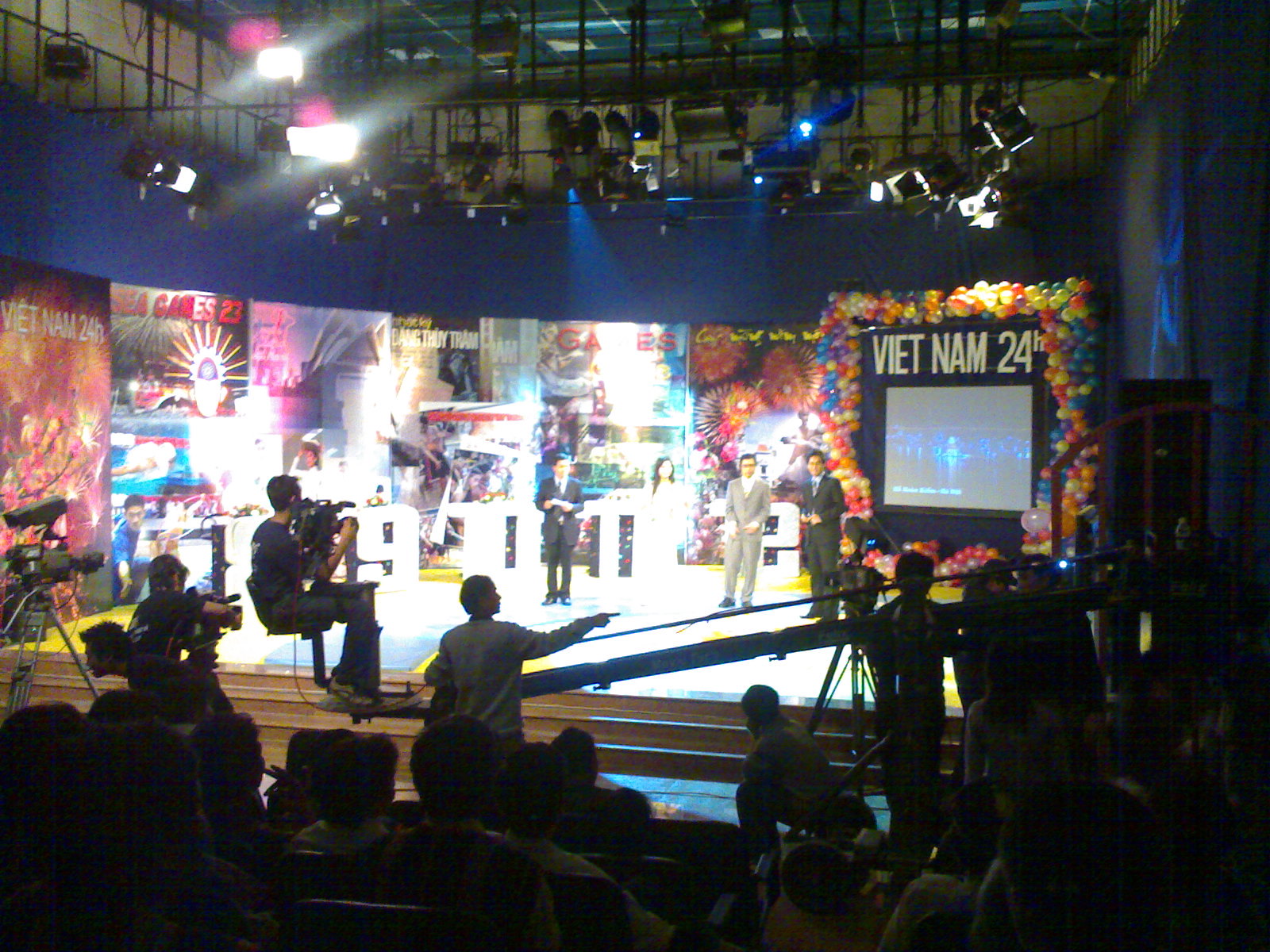The photograph, a full-color albeit poor-quality image, captures a bustling television studio set during a live production. Overhead, the studio ceiling brims with bright spotlights flooding down onto the set, which is dominated by vivid multicolored decorations. Central to the scene is a prominent display featuring the text “Vietnam 24,” surrounded by a blue border and a cluster of vibrant balloons. The display seems to incorporate a video monitor. 

On stage, there are four people, including a host in a tan suit, another in a black suit, and possibly a female host in a business skirt suit. The backdrop behind them showcases an array of colorful posters, contributing to the festive or commemorative atmosphere. To the left, two cameramen are visible, along with a director who is pointing towards someone off-screen.

An audience sits in shadows at the bottom of the image, all eyes directed toward the stage. The set is alive with colors—white, black, pink, blue, green, orange, yellow, gray, silver, and purple. The setting suggests a celebratory or memorial event related to “Vietnam 24,” potentially commemorating a significant anniversary or event.